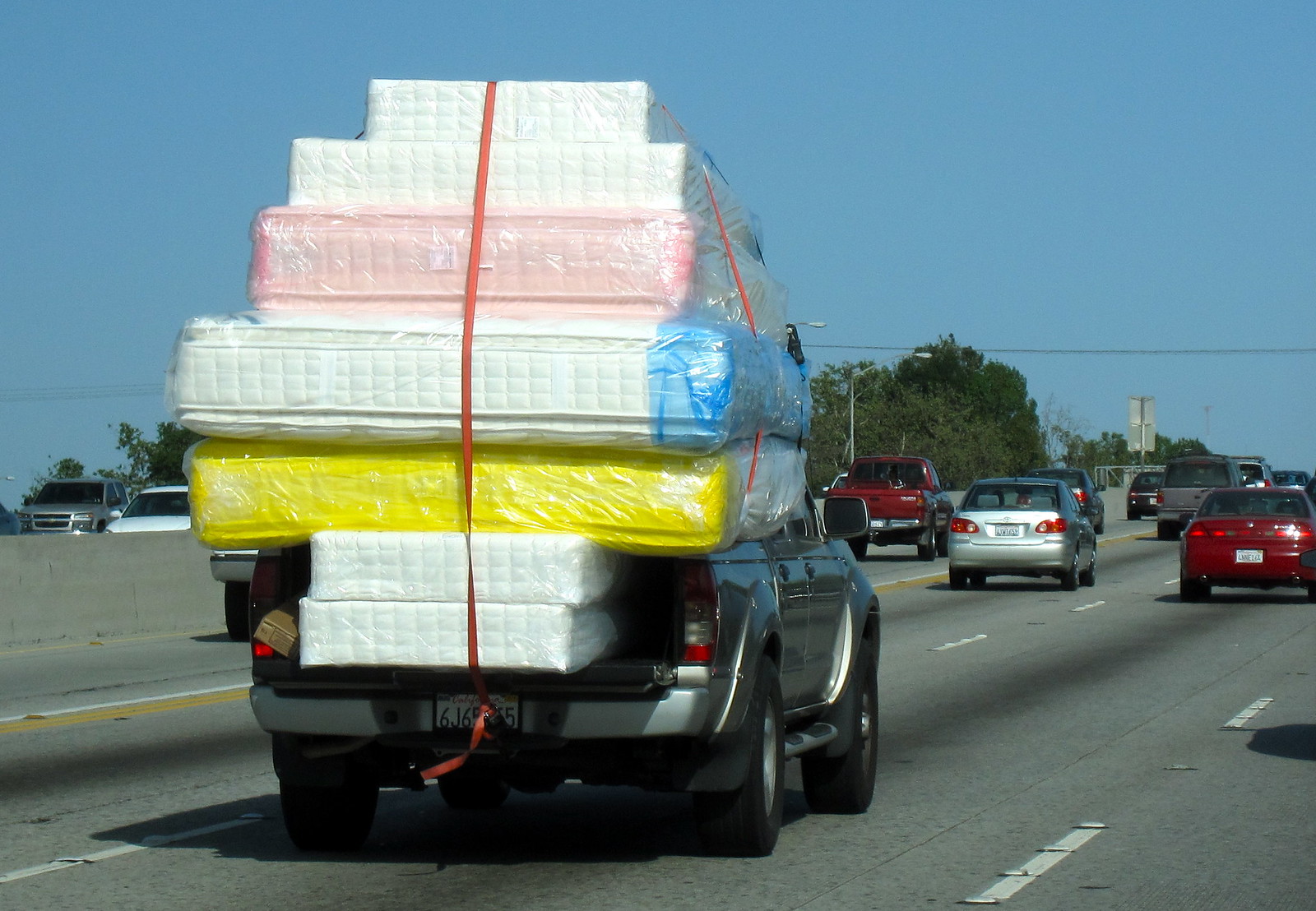This photograph captures a precarious scene on a European motorway, where a silver pickup truck with a white license plate, partially visible as “6J6”, is transporting a concerning load of mattresses. The vehicle is traveling in the third lane of a four-lane highway, and the image is taken from the fast lane to its left. Stacked high in the open bed of the pickup are seven mattresses of varying sizes and colors, ranging from twin to king size. Specifically, the back contains two small twin-sized mattresses at the bottom, a king-size mattress wrapped in yellow, another large white mattress with a quilted border partially wrapped in blue plastic, a smaller mattress in pink wrapping, and finally two additional white mattresses of decreasing sizes at the top. The mattresses are secured, if precariously, with three red ratchet straps arranged haphazardly around the load. Other vehicles can be seen on the clear, sunny motorway, suggesting the driver and surrounding passengers may have more at stake than meets the eye. This dubious transport method raises safety concerns, as the load appears unstable and risky for other road users.